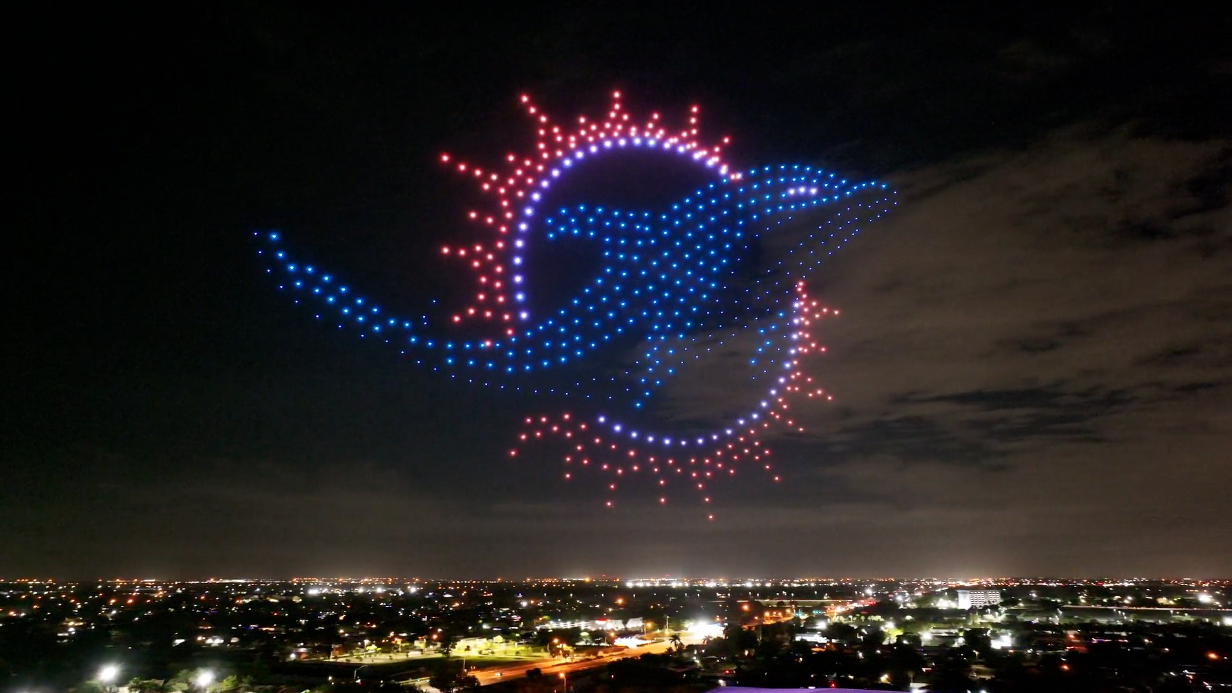This nighttime cityscape photograph captures a lively metropolis illuminated by myriad lights at the bottom fifth of the image, predominantly showcasing a dark, slightly cloudy sky. Above the city, an awe-inspiring display features a dazzling formation that appears to be created by either fireworks or a high-tech drone show. The spectacle in the sky resembles a majestic crown-shaped arrangement of lights, predominantly orange and white, through which a vividly detailed blue dolphin—complete with visible fins, tail, and a white eye—seems to be diving. This ethereal dolphin appears to emerge through the center of the crown-shaped lights. The dolphin's upward-facing tail and head give the impression it is leaping through this ring of lights, accentuated by a red sunburst design with a small blue circle at the center hovering above it. The intricacy and precision of the display evoke a sense of wonder, suggesting an advanced, possibly AI-generated visual experience. Below, you can discern architectural structures, streets, and businesses, along with a highway slicing through the illuminated urban sprawl, grounding the fantastic aerial display against the backdrop of everyday urban life.